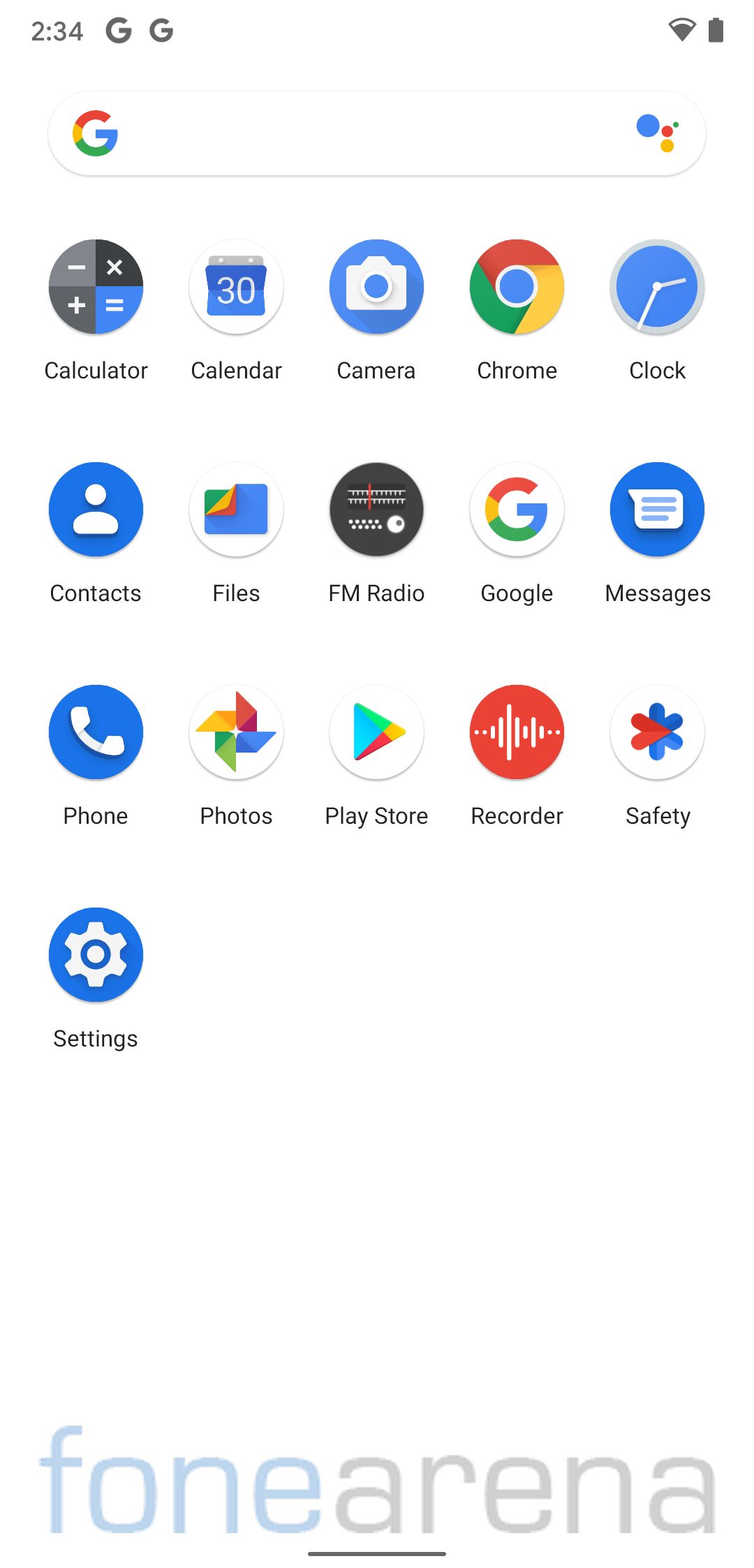The image depicts a close-up of a phone's home screen. At the top left, the time displays "2:34" alongside two "G" symbols, with one slightly larger than the other. On the right side of the top bar are indicators for Wi-Fi and battery status. Below this is a white, oval-shaped Google search bar featuring a "G" logo on the left side, and four dots in blue, red, yellow, and green on the right.

Beneath the search bar are neatly arranged icons corresponding to various apps, organized into rows. Here's the detailed layout:

1. **First Row**: 
   - Calculator (black, gray, and blue with white accents)
   - Calendar
   - Camera
   - Chrome
   - Clock

2. **Second Row**: 
   - Contacts
   - Files
   - FM Radio
   - Google
   - Messages

3. **Third Row**: 
   - Phone
   - Photos
   - Play Store
   - Recorder
   - Safety

4. **Fourth Row**: 
   - Settings

At the very bottom of the screen, a label reads "FoneArena" (spelled as "F-O-N-E-A-R-E-N-A" in segmentation), with "Fone" in blue and "Arena" in light gray. A thin light black line runs underneath this label. Notably, there is a substantial white space below the last app icon and above the "FoneArena" label, giving the screen a clean and organized appearance.